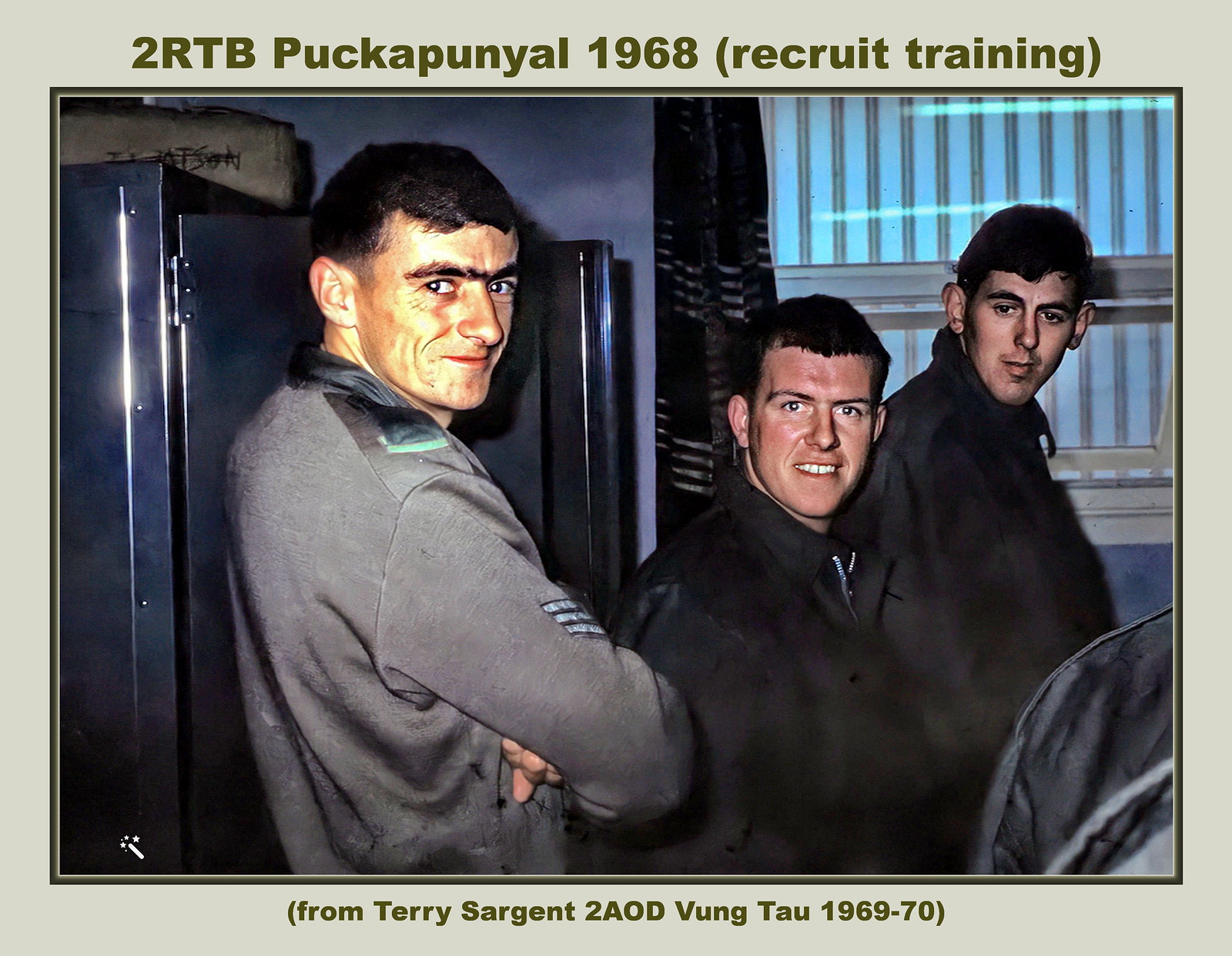The photo is a color image from 1968, featuring three smiling men with black hair, white complexions, and military uniforms, each bearing insignia. The man in the foreground on the left is leaning against a few gray lockers, looking over his right shoulder with his arms crossed. The other two men, likely new recruits, stand to the right, both wearing black zip-up jackets. Behind them, there is a window adorned with plaid curtains, possibly black or blue, and a structure visible outside. The image is set within a light olive-green border, with dark green text at the top reading "2RTB Puckapunyal 1968 (Recruit Training)" and at the bottom "From Terry Sergeant to AOD Vung Tau 1969-70."